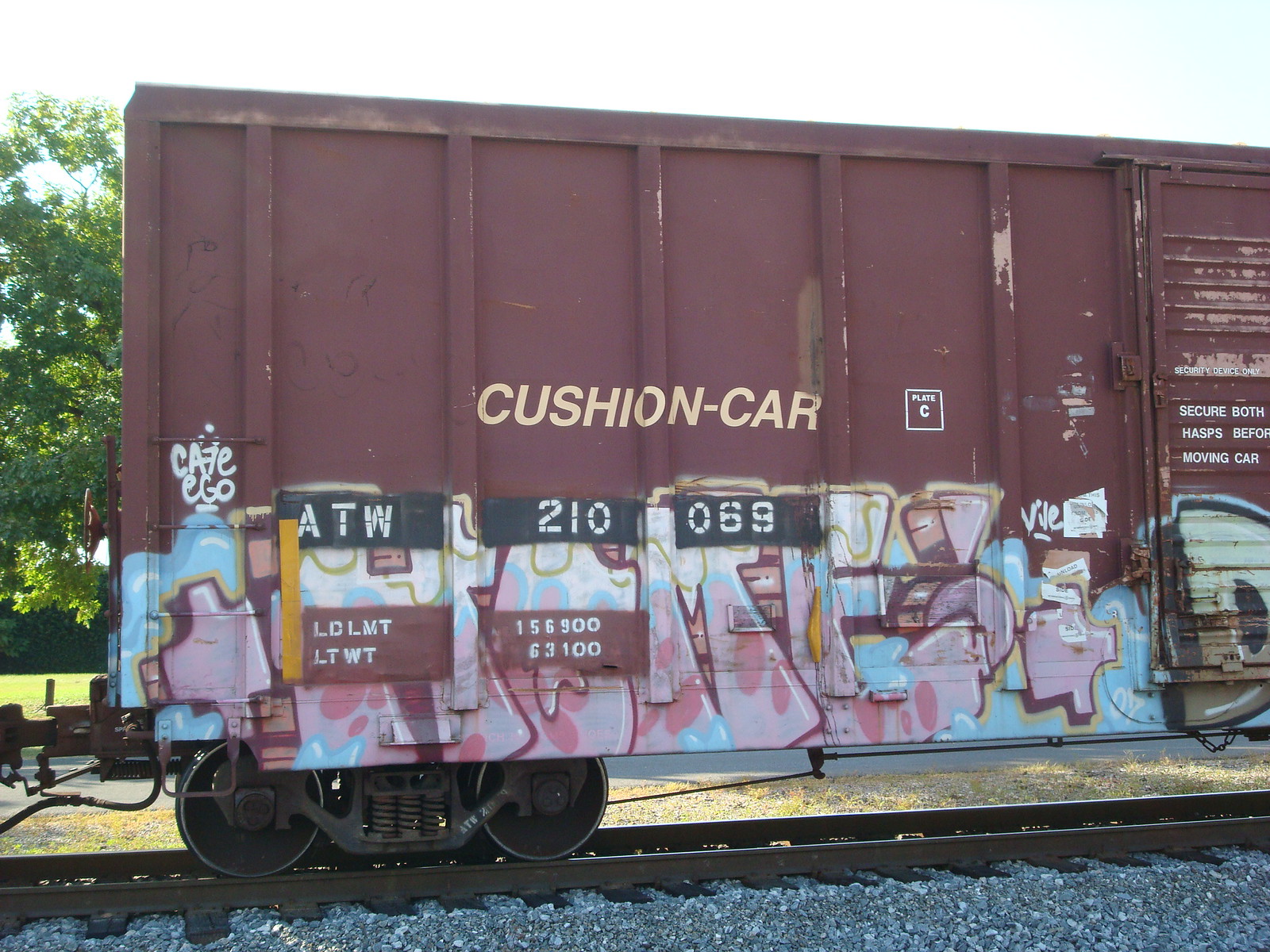This photograph captures a detailed side view of a maroon-colored train car, resting on the tracks with the familiar rocky gravel beneath it. The bright midday sun casts distinct shadows between the train car and the rails, enhancing the vividness of the scene. The train car, stamped with "Cushion Car" and marked "ATW 210 069" along with other serial numbers and instructions like "LCLM TLT WT 156900," exhibits wear with patches of peeling paint and rust. Covering parts of the car is graffiti in shades of light pink, white, and blue, resembling puzzle pieces with some indistinguishable markings. To the right side of the car, there is a sliding door and a cautionary note that reads "Secure hasps before moving car." Beyond the tracks, a grassy field stretches out with trees framing the background under a bright sky. The train car dominates the photograph, with no other cars visible in the frame.